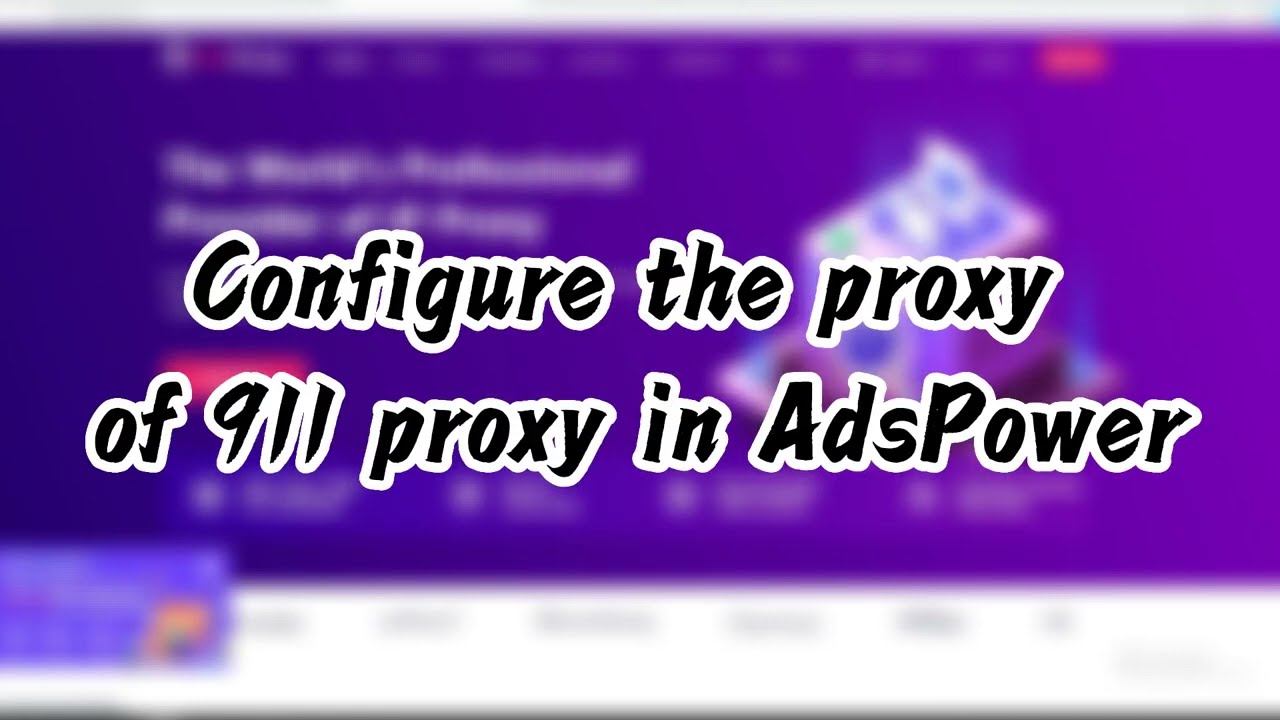The image primarily features a purple and blurred background, creating a somewhat indistinct view that resembles a screenshot of a website or a presentation slide, perhaps displayed in PowerPoint. Prominently positioned in the center of the image is two lines of text, framed by a white outline with black lettering that reads, "configure the proxy of 911 proxy in Ads Power." Additionally, there's a white rectangular strip spanning the width of the lower portion of the image, along with a small purple rectangular panel extending from the lower left side. Despite the blurriness, various colors such as purple, gray, white, black, yellow, orange, green, blue, and even hints of red add to the overall colorful composition.